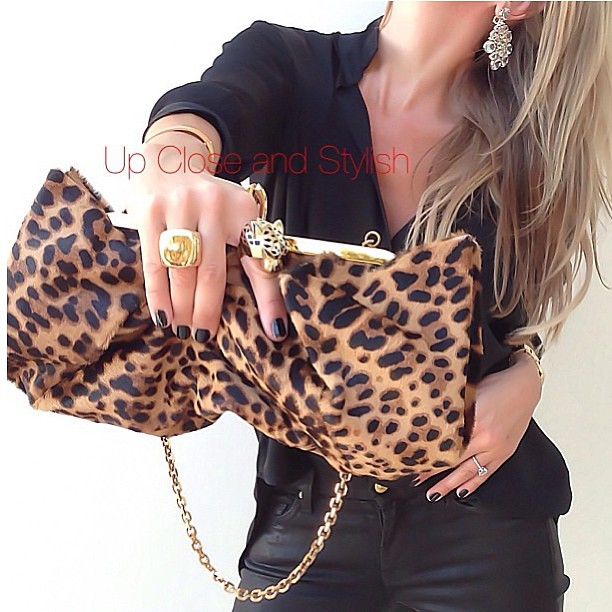This image, likely an advertisement for a fashion brand, showcases a woman from the neck down to the upper thigh, emphasizing her attire and accessories. She has long, wavy blondish hair cascading from the top right corner of the frame. Her left ear is adorned with a large, tear-drop-shaped silver earring. She is dressed in a black v-neck shirt paired with tight-fitting black leather pants. Her right arm extends toward the camera, prominently displaying a leopard print purse with a gold chain handle. The purse is a beige color with black polka dots, reminiscent of a cheetah design. The top of the purse is gold, matching the chain. Her nails are painted black, and she wears a large, square gold ring on her right ring finger and a yellow leopard-patterned ring on her pointer finger. There is a red overlay text in a narrow font that reads "up close and stylish."